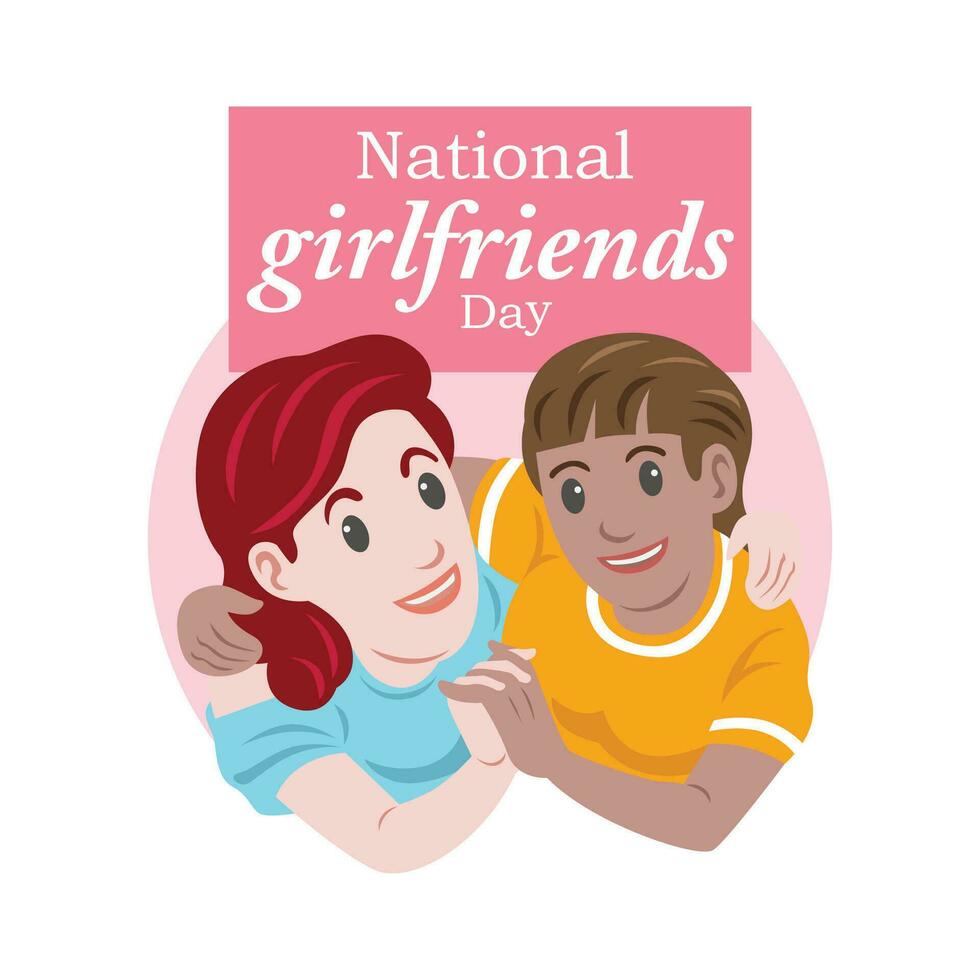This colorful cartoon poster celebrates National Girlfriends Day with a prominent pink rectangle at the top that contains the event's name. "National" appears on the first line in a Chimes New Roman type font, while "girlfriends" is italicized and bolded in white letters, followed by "Day" in all caps. Below this, a pink circle serves as the background, partially cut off at the bottom by two women embracing each other. The woman on the left has shoulder-length, curly red hair, red eyebrows, black eyes, and light skin. She wears a turquoise short-sleeved shirt and is smiling, showing rose-colored lips and her teeth. Her arm is wrapped around the woman on the right, who has short brown hair, brown eyebrows, greenish eyes, and slightly darker skin. The woman on the right is wearing an orange short-sleeved shirt with white trim around the neck and sleeves. Both women are smiling at each other, their arms around each other's shoulders, and their free hands clasped together in front of them.